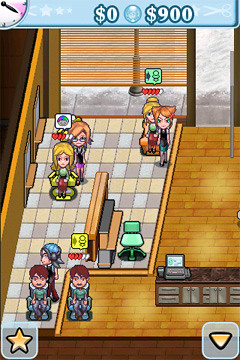This image is a detailed screenshot from what appears to be a mobile game set inside a cartoon-styled office or possibly a hair salon or diner. The scene is vibrant with multiple characters, both male and female, scattered around the room. Some of the characters are seated in chairs and in front of mirrors on the left-hand side, while others stand or move about the room. The floor is divided into a checkered tile pattern on the left and a laminate brown on the right. Above the characters, small icons, including hearts, give additional context or status for the characters. 

At the top of the image, a light blue UI bar displays $0 and $900 alongside a clock icon. There is a laptop on the counter near the bottom of the image, and additional game UI elements are present: a star button at the bottom left and a downward-pointing arrow at the bottom right. This blend of interactive elements and detailed environmental setup creates a lively and engaging scene typical of simulation mobile games.